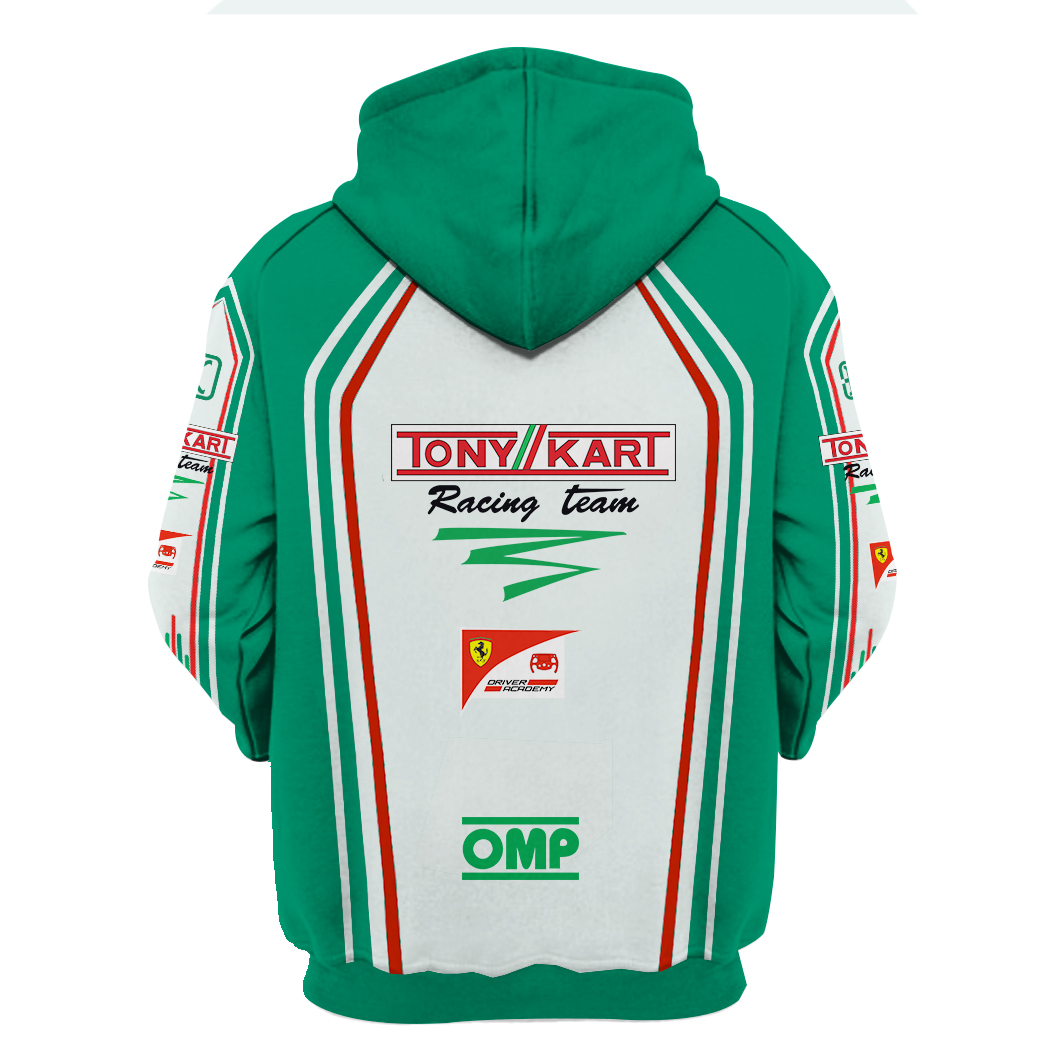The image depicts the back view of a green hoodie associated with the Tony Kart Racing Team. The hoodie features a prominent white design on the back, shaped somewhat like a tombstone. Within this design, the words "Tony Kart Racing Team" are boldly displayed in red text. Beneath these words, there’s a sequence of lines in the colors of the Italian flag: green, white, and red, mimicking Italy's national colors. Additionally, the design includes a zigzag figure and partially visible lettering, suggesting sponsorship details, though some are too blurry to decipher fully. The bottom of this white design section is marked with the acronym "OMP" in green, flanked by green lines above and below it. This OMP branding is also repeated on the green and white sleeves, maintaining consistency in the overall design elements seen on the hoodie.